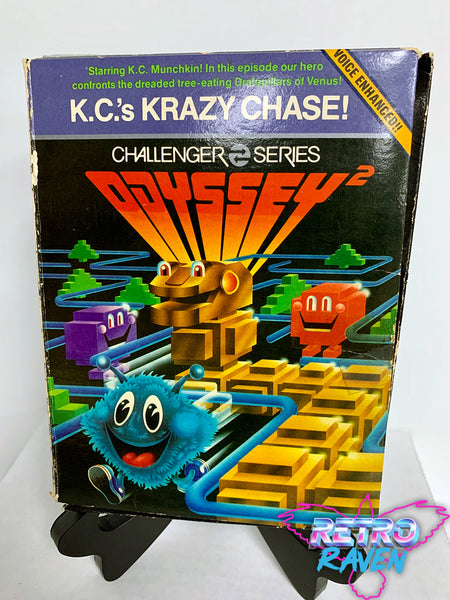The cover image for Casey's Crazy Chase, part of the Challenger Series for Odyssey 2, is predominantly rendered in purple and black hues. Central to the design are four distinct characters: a fuzzy, blue, happy-faced creature that looks like an anthropomorphic animal, running energetically through a maze; and three chasers – an orange monster, a gold robot, and a purple monster, all with smiling faces. The top section of the cover features a blue rectangle with the text: "Starring Casey Munchkin. In this episode, our hero confronts the dreaded tree-eating Droletors of Venus." Below it, the title "Casey's Crazy Chase" is prominently displayed in white text, alongside "Challenger Series" in capital letters. The branding "Odyssey 2" appears in striking orange text. Notably, in the lower right-hand corner, "Retro Raven" is inscribed in blue letters. This vibrant and detailed cover art effectively encapsulates the adventurous and whimsical essence of the game.